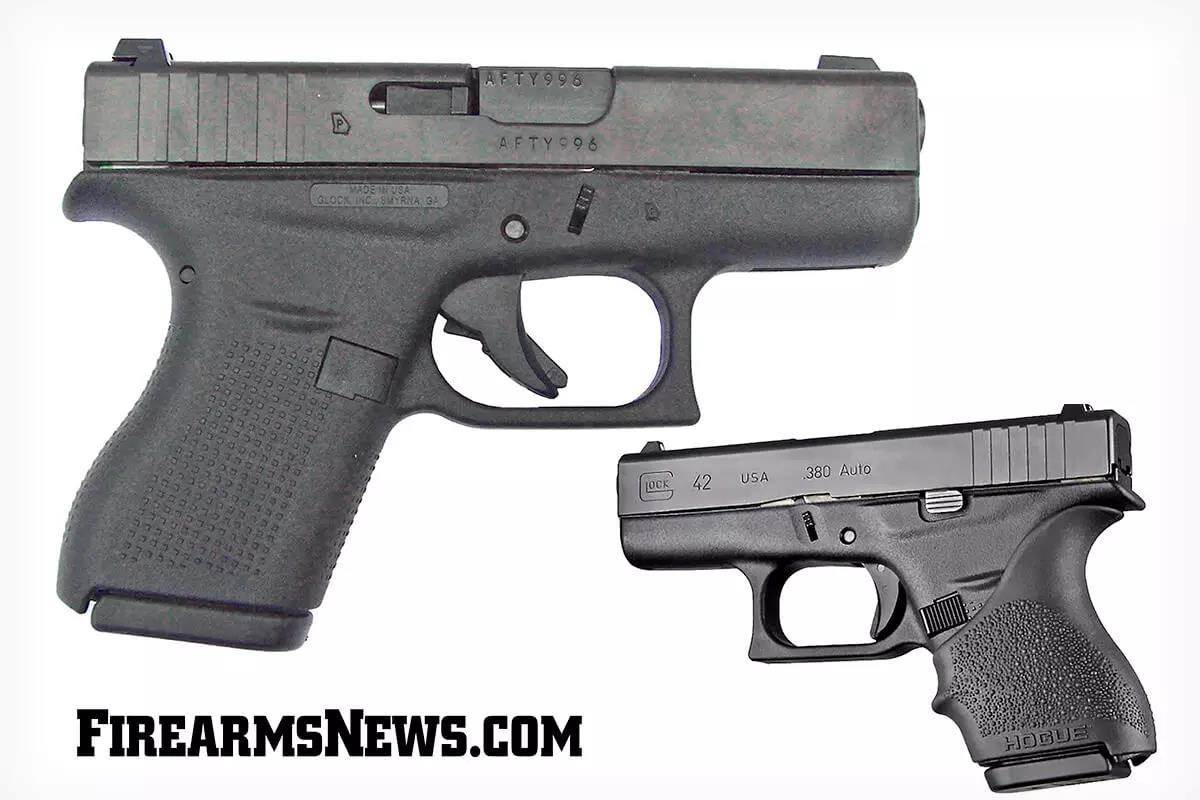The image is a horizontally oriented rectangle with a white background. In the bottom left corner, it displays the text "firearmsnews.com" in black. The illustration features two handguns. The larger handgun in the top left corner is dark gray with a lighter gray slide, pointing to the right, displaying the right side. Markings on it include "AFTY-996" on the barrel and "Made in USA, Glock Incorporated, Smyrna, Georgia" on the handle. The smaller handgun in the bottom right corner, facing left and displaying the left side, features similar coloring with "HOGUE" written on the bottom of the handle. The top of this smaller gun reads "Glock 42 USA .380 Auto." Both handguns have a textured, grippy handle, and appear to be Glocks based on their design and markings.